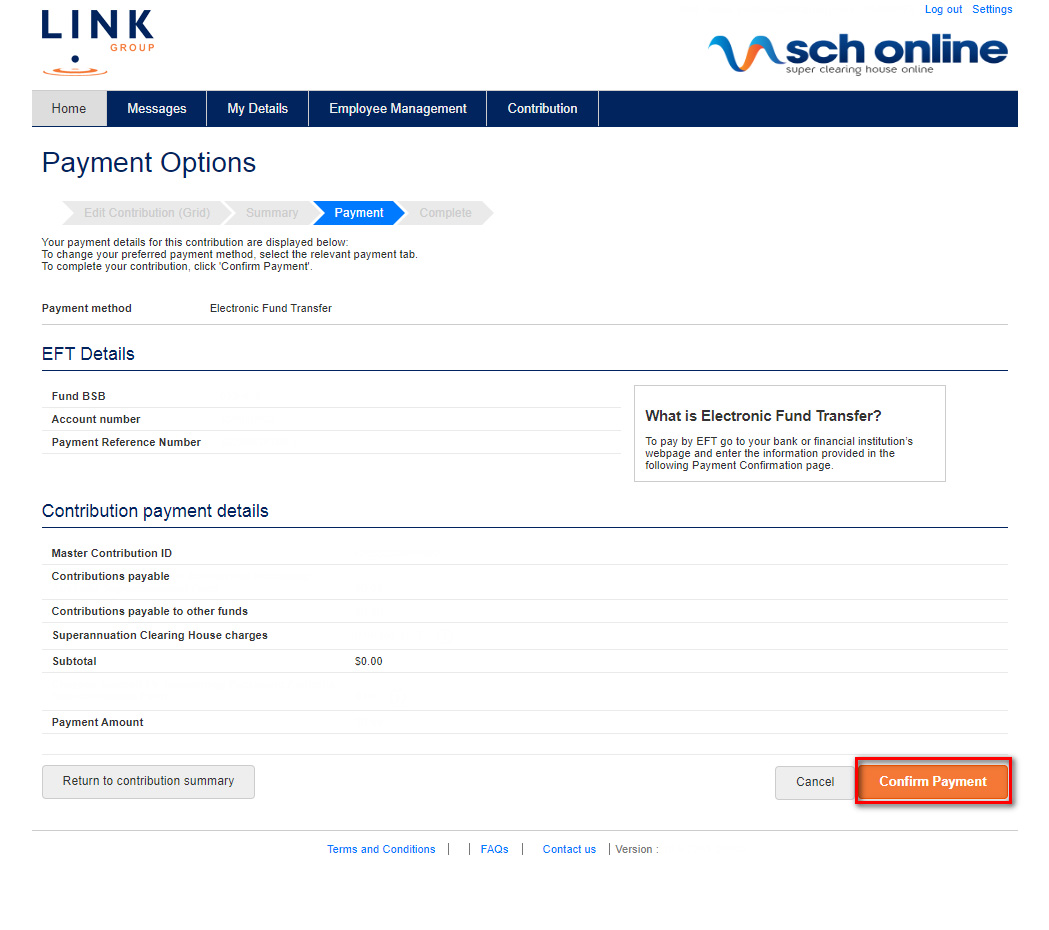Here's a detailed and cleaned-up descriptive caption for the given image:

---

The image depicts a webpage from a site called "SCH Online" featuring a user dashboard with various navigational and functional elements.

At the top-right corner, there is a "Logout" and "Settings" option. Adjacent to it lies a decorative blue squiggly line with an orange background accent. On the far left corner, the word "LINK" is prominently displayed in capital letters followed by the label "GROUP" in orange. Directly beneath this, there is an image of a ball creating a splash effect.

In the left sidebar navigation, the following options are listed:
- **Home**: Displayed with a gray button next to it.
- **Messages**: Highlighted in blue.
- **My Details**
- **Employee Management**
- **Contribution**

The main content area is focused on payment options. At the top, "Payment Options" is prominently displayed in blue text, followed by a list of steps indicating that the process is in the third or fourth step. There's a blue label reading "Payment," with a note stating users can change their payment information if needed. A section titled "EFT Details" follows, with labeled fields for "Fund BSB," "Account Number," and "Payment Reference Number."

To the right, there is an informational box labeled "What is Electronic Fund Transfer (EFT)?", providing instructions about entering the given information on a bank or financial institution's webpage to make a payment via EFT.

Further down, a header reads "Contribution Payment Details," under which are the following fields:
- **Master Contribution ID**
- **Contributions Payable**
- **Contributions Payable to Other Funds: Superannuation**
- **Annuation Clear House Charges**
- **Subtotal**: Displayed as zero.
- **Payment Amount**: A blank field.

At the bottom of the page, there are three options:
- **Return to Contribution Summary**: A gray button.
- **Confirm Payment**: A conspicuous orange button with a red border, located all the way to the right.
- **Cancel**: A gray button located to the left of the "Confirm Payment" button.